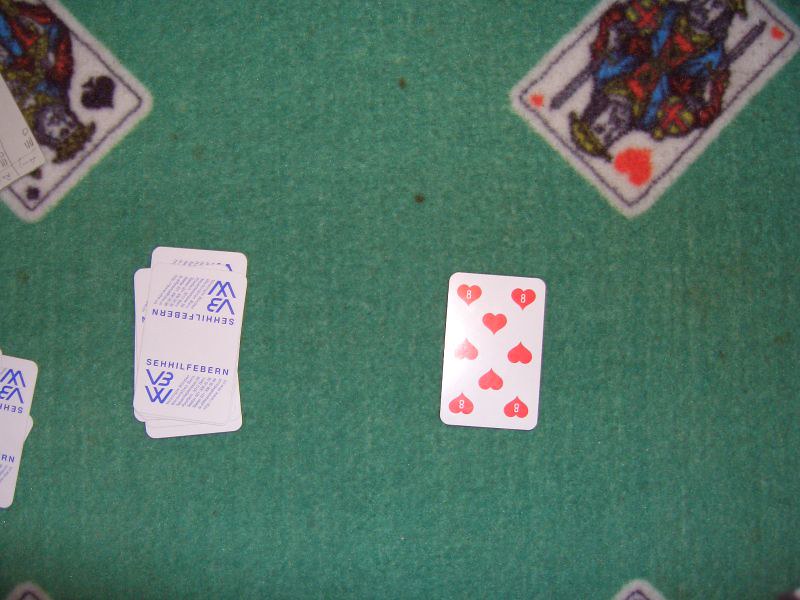The image captures a well-worn playing card table covered in green felt. Each corner of the table is adorned with artwork depicting playing cards, including the King of Hearts and the King of Spades. On the table's surface, five playing cards are visible. Prominently, an eight of hearts card lies face up. To the left of the eight of hearts, there are three playing cards face down, positioned in the left-hand third of the image, while another two cards lie face down further to the left. The backs of these cards feature text that reads "S-H-H-I-L-F-E-B-E-R-N," along with additional characters "B," "3," and "W." The lighting comes from above, casting a noticeable reflection on the eight of hearts. Although the picture isn't sharply focused, the worn state of the table is evident, hinting at its frequent use.